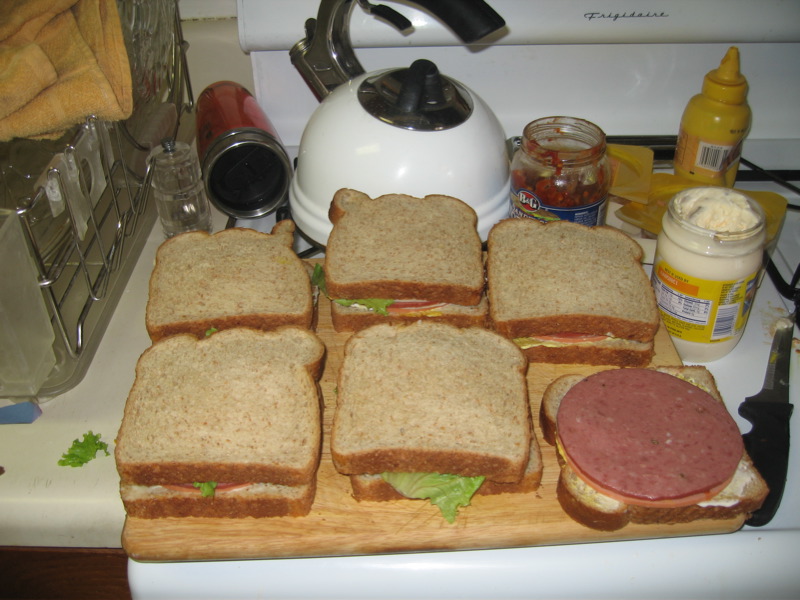The image shows a cluttered kitchen scene featuring a white Frigidaire oven topped with a light-colored, wooden cutting board that fits perfectly atop the stove. On the cutting board are six sandwiches arranged in two rows of three. Five of these sandwiches are fully made, with wheat bread that has a brownish tint, visible layers of bologna or salami, lettuce protruding from the edges, and hints of mayonnaise or mustard. However, the sixth sandwich in the lower right corner is open-faced, showing just a single slice of bread topped with two pieces of bologna.

In the background, an open jar of mayonnaise is visible to the right, a dirty knife with mayonnaise on the tip lies nearby on the oven, and an open jar of mustard can be seen in the upper right corner. Next to the mustard is an open jar containing a red spread, potentially salsa or something similar. A white and black metal teapot and a glass pepper shaker are also on the stove. To the right, beside the oven, sits a countertop that is cream-colored, with a metal dish rack on it, holding a yellow towel. A red thermos mug is laying on its side, adding a final detail to the busy kitchen setting.